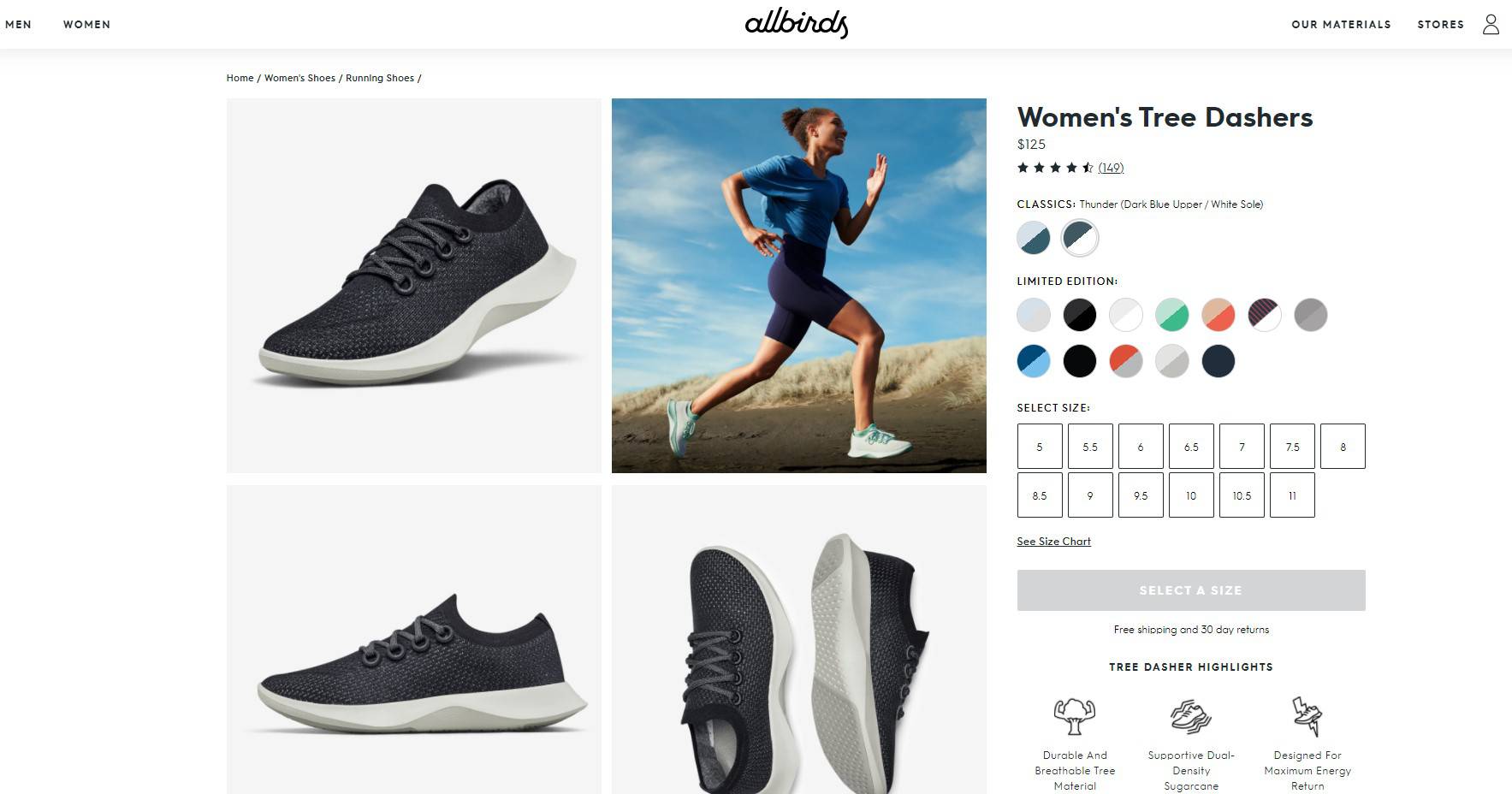This is a detailed screenshot of an apparel website focused on shoes. The header of the page prominently features the brand name "Allbirds" in large, black text. In the upper left corner, small black text lists the categories "Men" and "Women." On the right side of the header, additional links include "Our Materials," "Stores," and a profile icon for account management.

Directly below the header, the navigation path reads "Home / Women's Shoes / Running Shoes," indicating the current category the user is viewing. The main section of the page displays four images. The top left, bottom left, and bottom right images showcase a pair of dark gray and black running shoes with white soles. The upper right image features a woman running, dressed in a blue shirt and navy spandex shorts, wearing similar shoes.

To the right of these images, there is a product description that reads "Women's Tree Dashers," priced at $125. The product has received a rating of four and a half stars. A variety of color options and sizes are available, ranging from sizes 5 to 11.